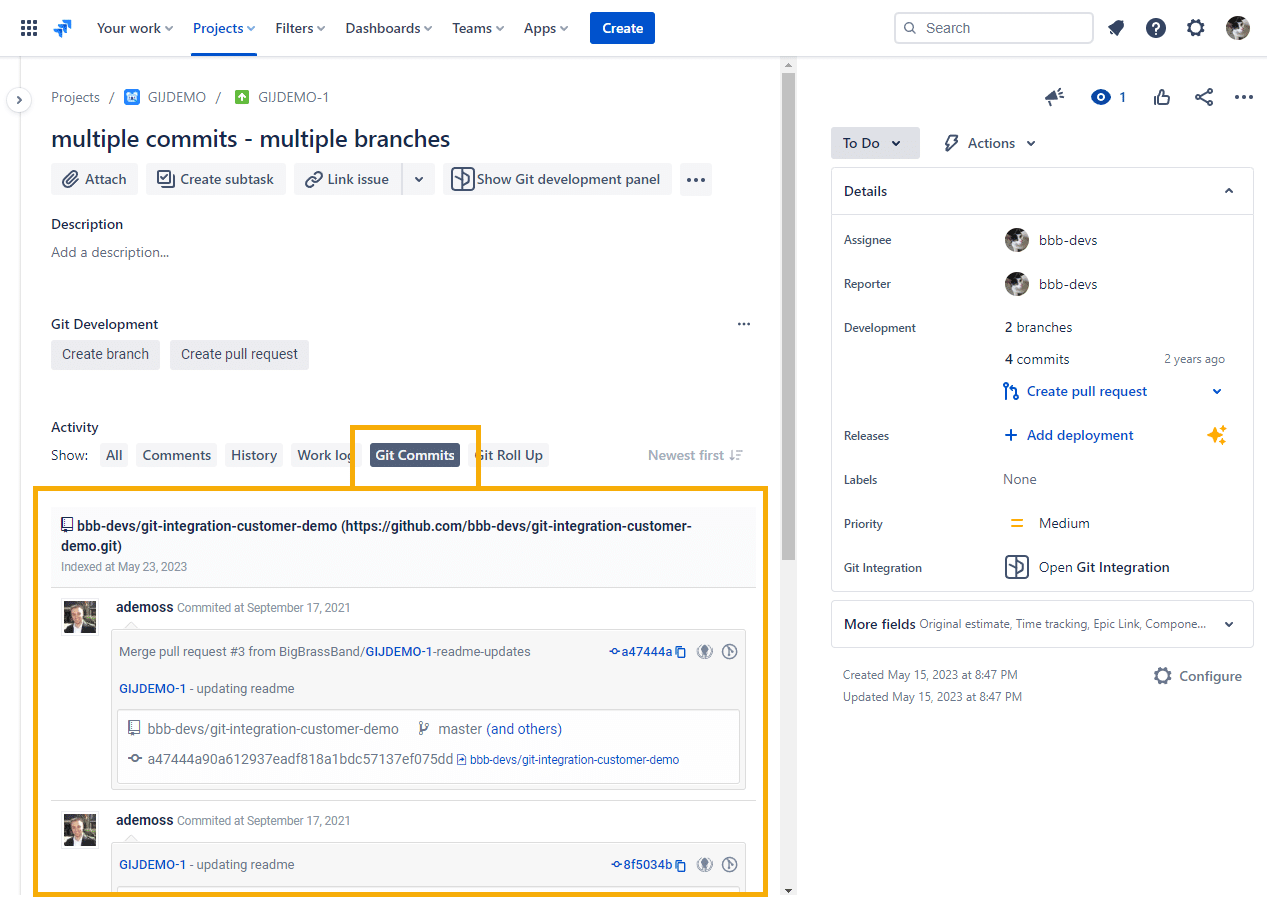In this screenshot, set against a pristine white background, we observe a detailed interface from what appears to be a project management or development platform. 

**Top Right Corner:** 
- A circular icon featuring an image of a tuxedo cat.
- Icons for Settings, a Help icon denoted by a question mark within a black circle, and a bell icon for notifications.

**Top Left Section:**
- Menu items labeled as: "Your Work," "Projects," "Filters," "Dashboards," "Teams," and "Apps."
- A prominent blue button labeled "Create."

**Directly Beneath the Menu:**
- Written in bold black text: "Projects" followed by project names "GidgeDemo" and "GidgeDemo1."

**Left Sidebar:**
- Text options for "Multiple Commits" and "Multiple Branches."
- Functionality buttons for attach, create subtask, link issue, and show Git development panel.

**Main Content Area:**
- An orange-bordered rectangular box labeled "Git Commits."
- A social media-styled post from a user named Aadmos, committed on September 17, 2021.
- The post includes a small image of Aadmos, who is seen wearing a dark suit jacket and white shirt.
- The message reads: "Merge pull request #3 from Big Brass Band/GIDGETDEMO1, readme updates. GidgeDemo1 updating readme."

This detailed caption encapsulates the contents and layout of the interface, highlighting key areas and functionalities available within the screenshot.